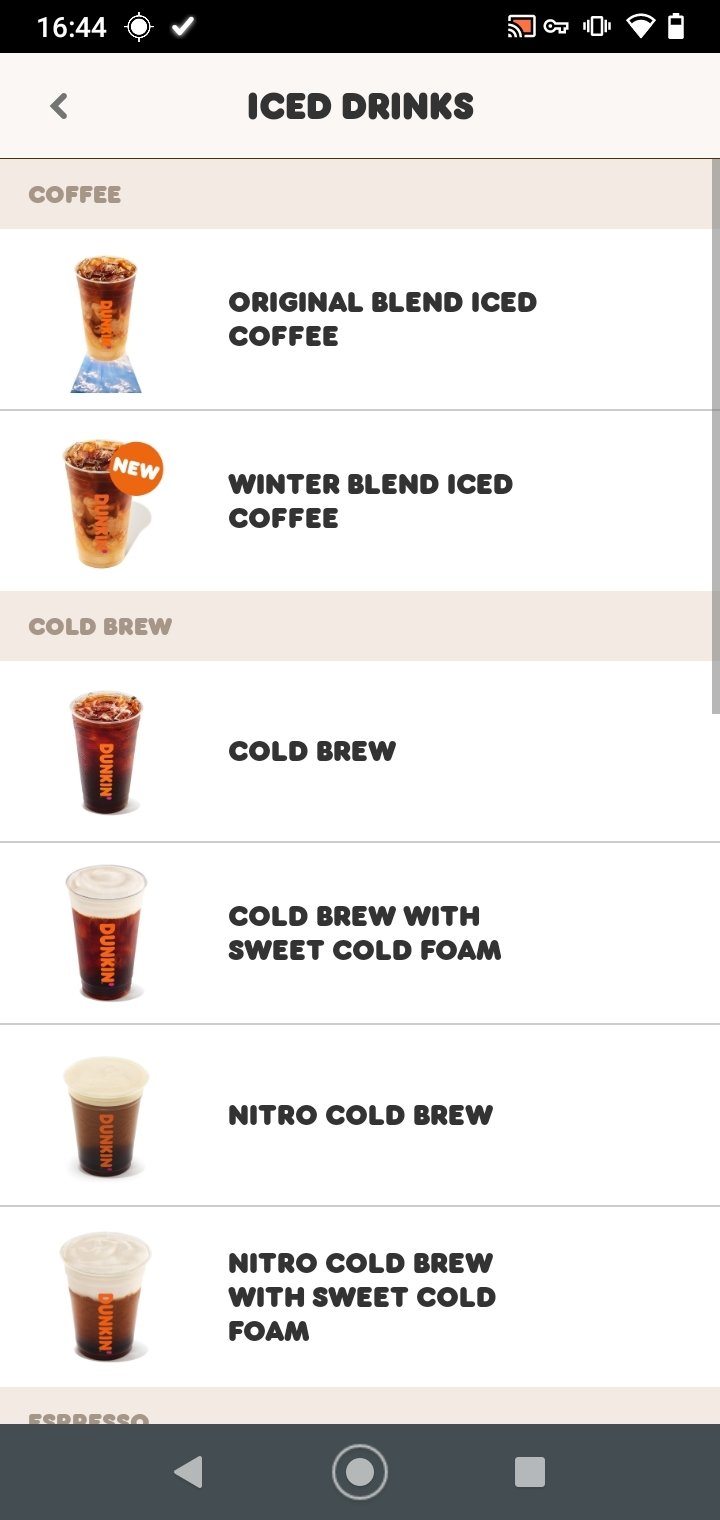This is a detailed screenshot from a Salfano tablet interface. At the top, there is a black strip displaying the time "16:44" in white text. Next to the time, there is a small circular icon with little points, which appears to be a location indicator. To the right of this icon, there is a white checkmark.

Moving further to the right, there is another icon for casting or sharing the screen to a TV, highlighted with an orange center. To its right is a key icon, followed by an icon indicating vibration mode (suggesting the sound is on vibrate). Next, there is a Wi-Fi signal icon, which looks a bit different from the usual Wi-Fi symbols. Finally, at the far right, there is a battery icon showing it is two-thirds full.

Below this top strip, there is a gray left arrow. In the center of the interface, the heading reads "Iced Drinks" in black text. The section starts with "coffee" and includes an image of a coffee cup. To the right of the image, it reads "Original Blend Iced Coffee."

Beneath this, there is a slightly larger image of a similar coffee cup with an orange circle containing the word "new" written in white. Next to this image, it states "Winter Blend Iced Coffee."

Following that, the section lists "Cold Brew" iced drinks:
- Cold Brew
- Cold Brew with Sweet Cold Foam
- Nitro Cold Brew
- Nitro Cold Brew with Sweet Cold Foam

Each of these drinks is accompanied by an image, all of which look very similar.